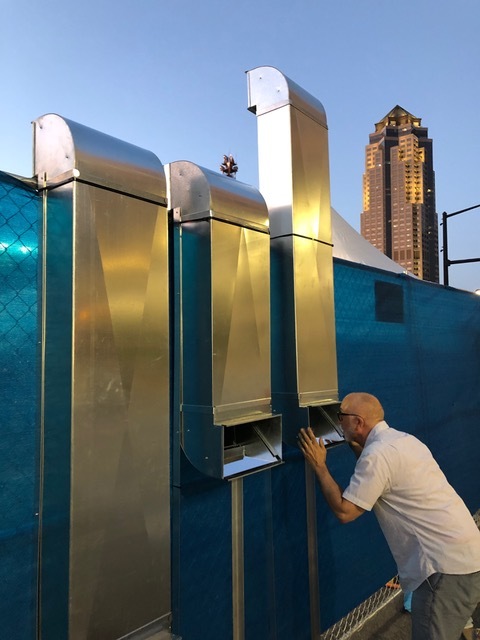This outdoor daytime photograph captures a bald white man with glasses, dressed in a white shirt and gray pants, standing in front of a blue wall. Attached to the wall are at least three tall, metallic periscopes, allowing the man to see over the wall. He's intently looking through the bottom of one periscope, which protrudes above the wall to presumably give him a view of a construction site behind it. The wall appears to be part of a chain-link fence covered with a blue tarp. In the top right corner of the image, a skyscraper with a gabled roof is visible against a clear, blue sky. The overall setting is urban with a mix of industrial and metropolitan elements, emphasizing the contrast between the periscopes and the surrounding cityscape.